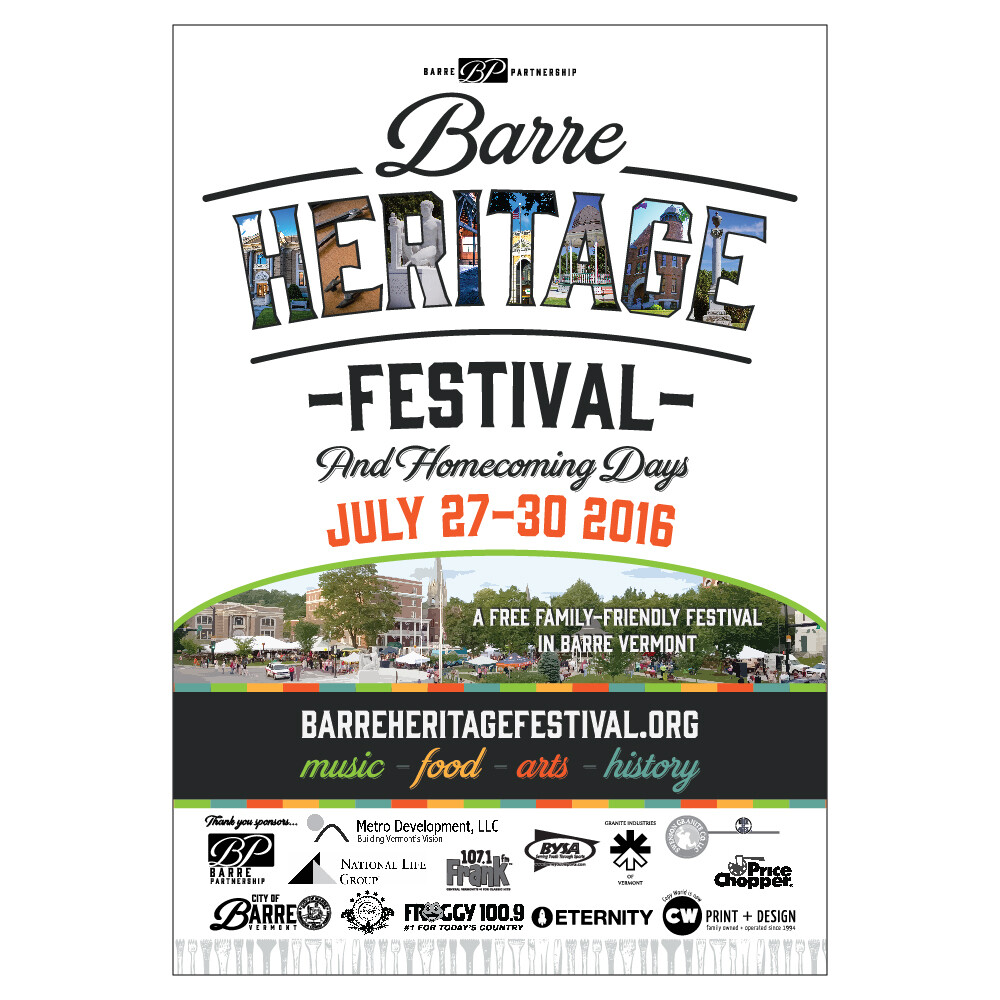This poster, predominantly white with graphic elements, advertises the Bari Heritage Festival and Homecoming Days, held from July 27th to 30th, 2016, in Bari, Vermont. Billed as a free family-friendly festival, the event's main attractions—Music, Food, Arts, and History—are highlighted in colorful text. The midsection features a city scene with numerous tents, embodying the festival atmosphere. Along the bottom are various sponsor logos. The festival's website, barheritagefestival.org, is prominently displayed, inviting attendees to learn more.